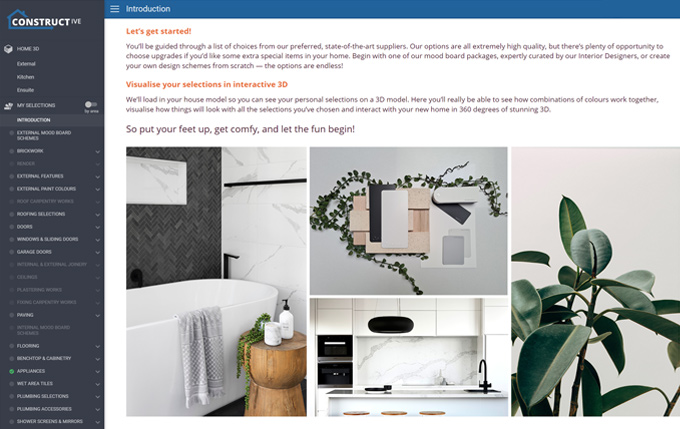The image depicts a detailed webpage or application interface with a clean, minimalist design. Thematically, the page has a white background with burgundy-colored text. On the right side of the screen, there is a gray-painted section featuring white text. 

At the top, a blue bar with white text reads "Introduction." Below this, the main white page displays burgundy text with an eye-catching message in yellow or orange that says, "Let's get started!" The subsequent burgundy text outlines the user journey, stating: “You'll be guided through a list of choices from my preferred state-of-the-art suppliers. Our options are all extremely high quality, but there's plenty of opportunity to choose upgrades if you'd like some extra special items in your home. Begin with one of our mood board packages expertly curated by our interior designers or create your own design scheme from scratch. The options are endless.”

The description continues to emphasize the interactive features: “Visualize your selections in interactive 3D. We'll load in your house model so you can see your personal selections on a 3D model. Here you'll really be able to see how combinations of colors work together. Visualize how things will look with all selections you've chosen and interact with your new home in 360 degrees of stunning 3D. So put your feet up, get company, and let the fun begin.”

Additionally, there are four images showcasing different interior spaces: a bathroom, a kitchen area, a top-down view of a room, and a close-up of a plant.

On the left side, within the gray-painted area, white text lists various sections including "Constructive Home 3D," "External Kitchen," "Enable My Selections," and "Introduction," among others, offering a structured navigation menu.